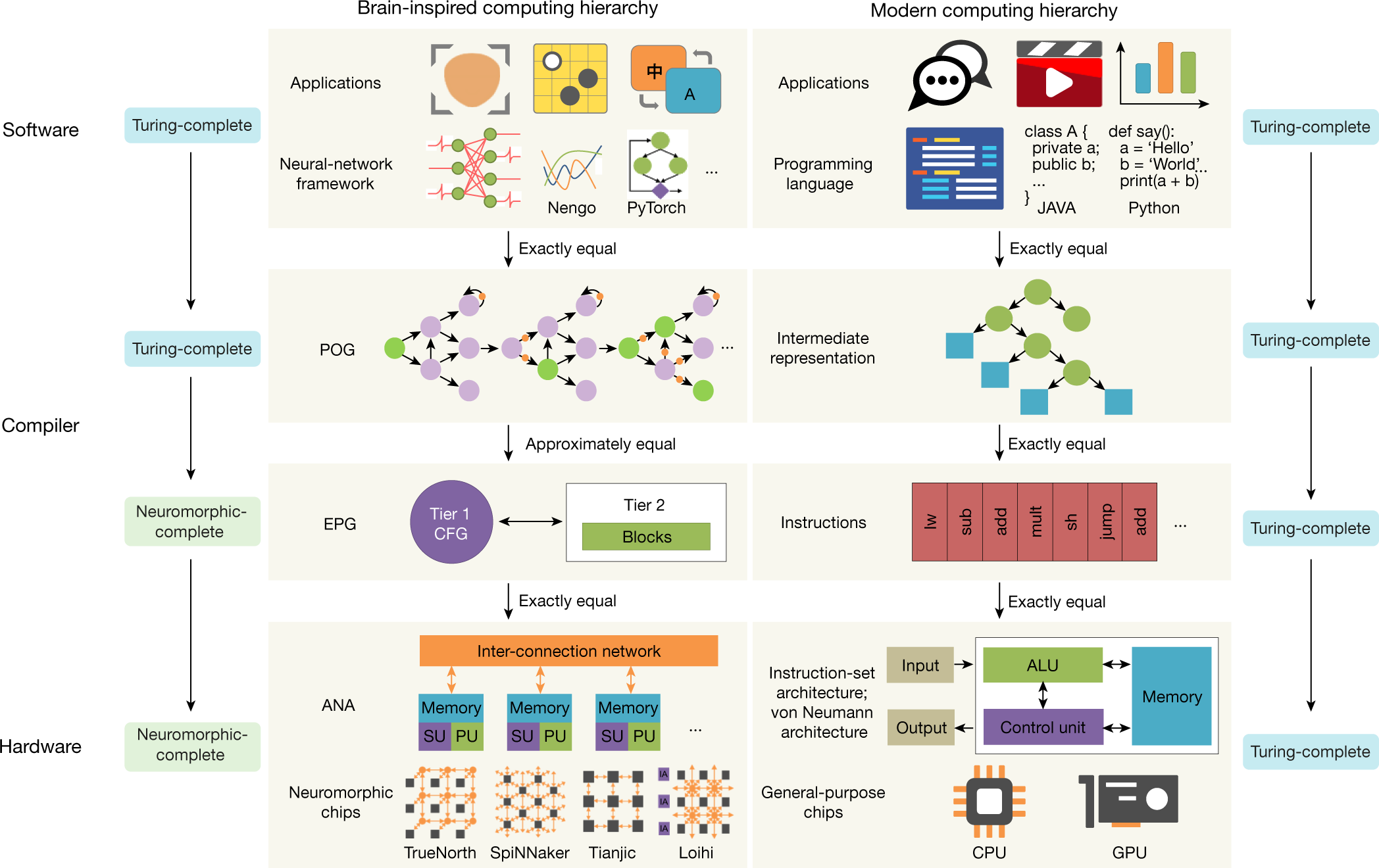This landscape image is a colorful, computer-generated diagram comparing the brain-inspired computing hierarchy to the modern computer hierarchy. The image features a detailed flowchart that spans various levels, illustrating the distinctions between the two computing paradigms. On the left side, it highlights key components such as software, compiler, and hardware, organized along the y-axis. The top section is titled "Brain-Inspired Computing Hierarchy," showcasing interconnected diagrams and icons labeled with terms like "application," "neural network," and "framework." On the right, corresponding elements of the "Modern Computing Hierarchy" are displayed. The diagram employs a vivid palette of oranges, blues, purples, and greens, with numerous arrows and labels to clearly delineate the pathways and functions within each hierarchy. Key terms like "Turing-complete" and "Neuromorphic-complete" are prominently featured, providing insight into the theoretical underpinnings of each system. The image is akin to a mind map, richly populated with icons and graphs that help visualize how computing processes are interconnected and function in both traditional and brain-inspired systems.